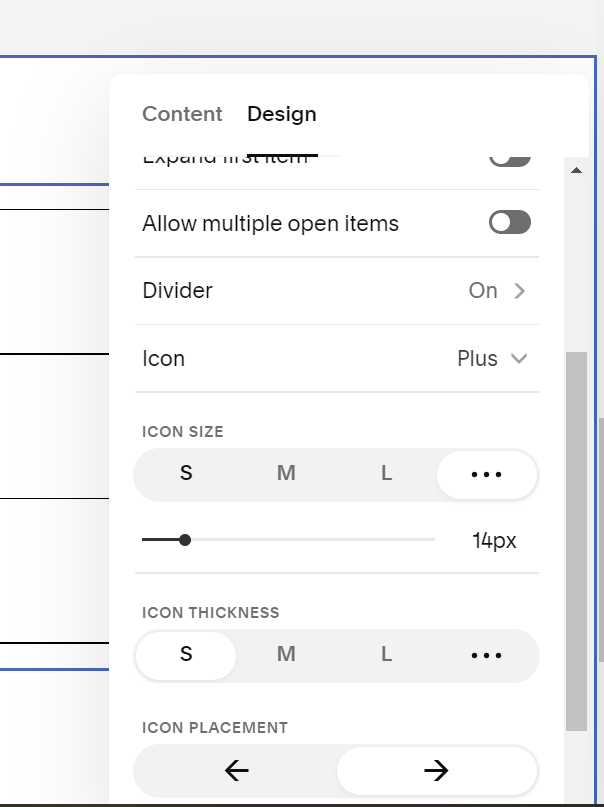A screenshot captures a user interface with a predominantly white background, interspersed with blue, gray, and black elements. The top of the image features a thin gray bar, followed by a blue line that wraps around one side. At the bottom, there's a thin black line. The interface consists of a white background with gray and black text.

At the top is a header labeled 'Content,' followed by 'Design,' which is underlined with a black bar. Below, a list of items is present:
- "Expand first item" with a corresponding black box and white circle.
- "Allow multiple open items," again accompanied by a black box with a white circle.
- "Divider on" with an arrow indicating further options.
- "Icon plus" with a direction arrow.
- "Icon size" inside a gray box, presenting size options S, M, and L. Below this, a white circle with black dots is visible.

Further down, a gray and black pull bar with a black circle and the text "14 px" appears. Another gray box below this offers size options (S, M, L) accompanied by three black dots. 

At the bottom, under the label "Bottom icon placement," another gray box contains two arrows: a black back arrow and a black forward arrow inside a white oval. To the side of the entire interface image is a visible gray scroll bar with an arrow.